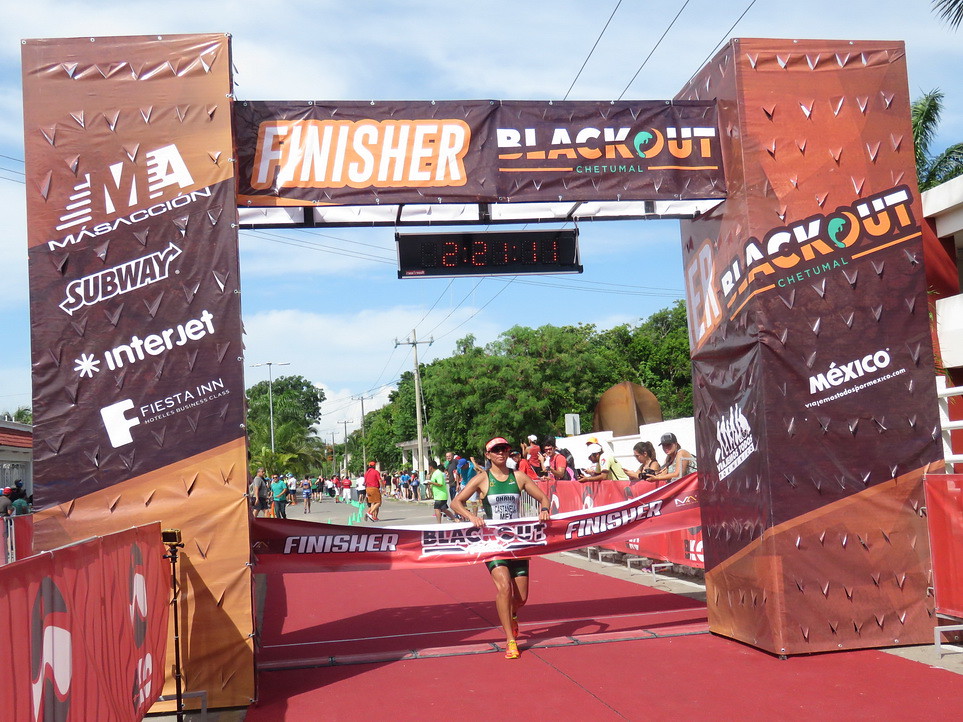The image captures the vibrant and momentous finish line of a triathlon, marked by a large arch adorned with various sponsor banners and logos, including Subway, Interjet, Fiesta Inn, and what seems to be references to Mexico. Dominating the scene is the word "finisher" prominently displayed, along with a digital clock below it reading 2:21:11 in red digits. A distinctive red carpet lines the finish area. In the foreground, a determined runner wearing a green top is about to cross the finish tape, while several spectators look on. The surrounding setting includes railings, cable lines, lush green trees, and the array of colors—green, black, red, white, brown, yellow, blue, and teal—offers a lively outdoor atmosphere. The event appears to be part of a series sponsored by Blackout Chitumo. This detailed and vivid scene blends the excitement of the race's climax with the presence of local and international backers.